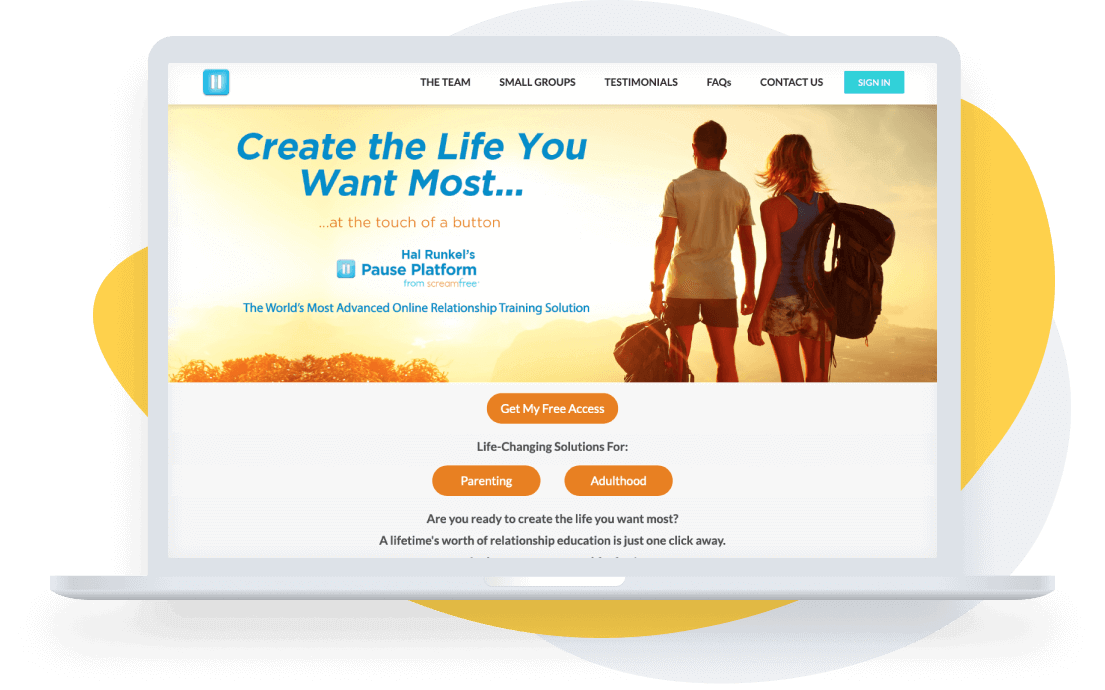A rectangular, landscape-oriented image with no clear borders, set against a white background, showcases a zoomed-in illustration of a laptop in the center of the frame. The laptop is depicted from a straight-on perspective, opened at a 90-degree angle, revealing only a sliver of its base where the keyboard would be, thus emphasizing its screen. The screen itself is roughly 30% wider than it is tall and has a light gray border along the top.

Behind the laptop, various irregular, ovular shapes in egg-yolk yellow and light gray extend beyond its boundaries, peeking out from the left, bottom, top, and right sides. These shapes create a dynamic backdrop for the central laptop image.

On the laptop screen, the webpage design is detailed starting with a white header in the upper left corner. A light blue box with two vertical white lines, resembling a pause button, is present. To its far right, a light blue rectangular field with the all-caps text "SIGN IN" in white is displayed. Adjacent to this, moving leftwards, are five more all-caps fields: “CONTACT US,” “FAQS,” “TESTIMONIALS,” “SMALL GROUPS,” and “THE TEAM,” which occupies about 35% of the way from the left side of the screen.

Below this header, a vibrant, sunshine-hued picture dominates the upper portion of the screen. It features two individuals from behind – a man on the left and a woman on the right, both clad in casual attire. The man, with broader shoulders and a thin waist, wears a white T-shirt, dark brown pants, and holds a backpack by his side. The woman, slightly behind him, dons a dark sleeveless top and patterned white shorts, with a large black backpack over her right shoulder. Her blonde hair cascades to her shoulders. Together, they gaze at a sunset.

To the upper left of these figures, italicized light blue text reads: “create the life you” followed by a line break and continuing with “want most...” Below, in orange font, it states: “...at the touch of a button.” Further down, in light blue, “Hal Runkles” is followed by “paws platform.” The phrase “paws platform” aligns next to the blue logo featuring a white pause symbol.

Beneath this picture, light blue text declares: “The world's most advanced online relationship training solution,” with each word initial-capped. The remaining bottom third of the image reverts to a white background, displaying three elongated, burnt orange ovals with rounded sides featuring:
1. Top center: "GET MY FREE ACCESS" in white text.
2. Below, split horizontally: "PARENTING" on the left oval and "ADULTHOOD" on the right oval.

Accompanying black text above the bottom ovals reads: “Life changing solutions for...” Below the bottom ovals, additional text queries: “Are you ready to create the life you want most,” followed by another line of text.